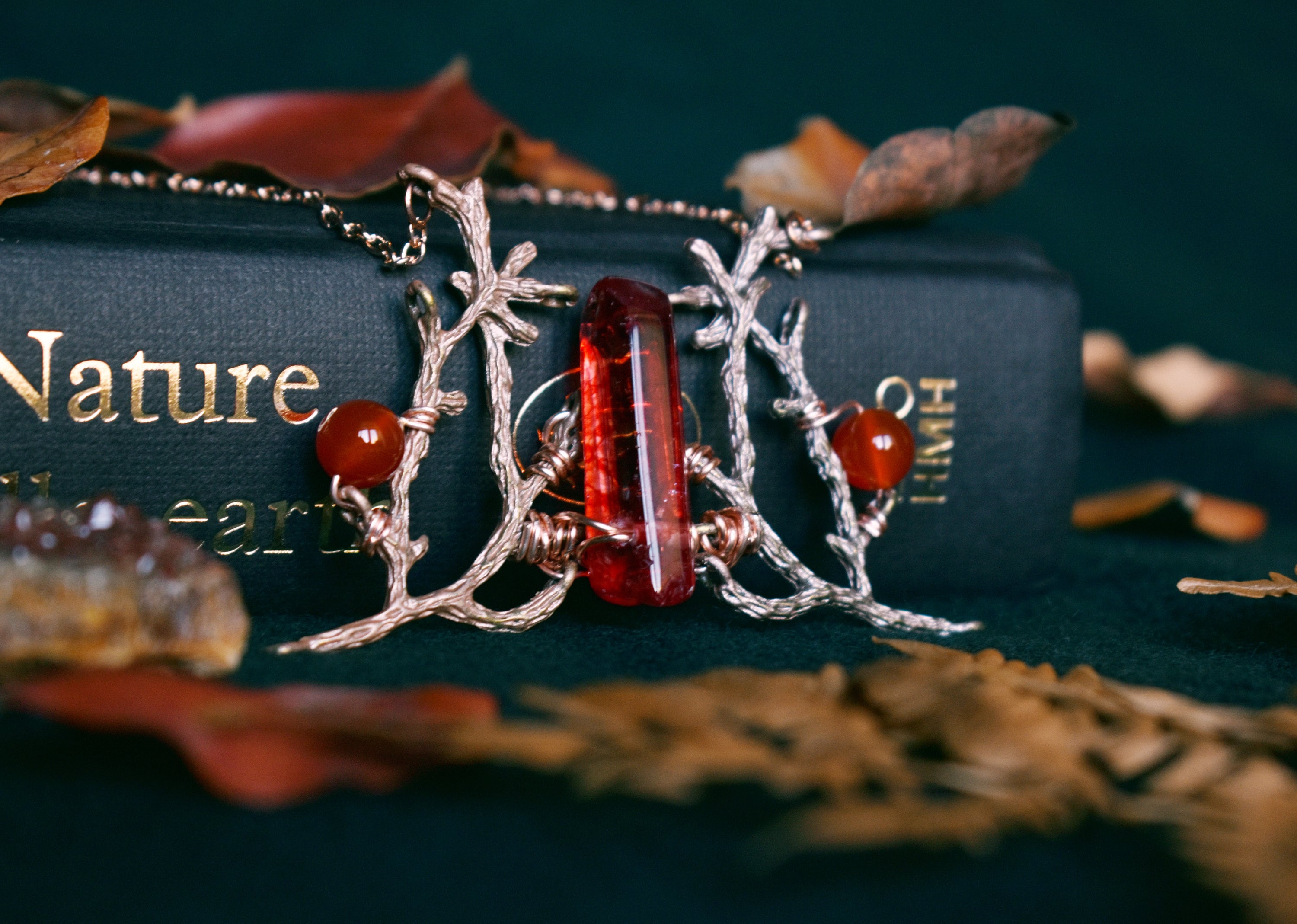In this detailed image, the focal point is a book with a black binding that prominently features the word "Nature" in gold lettering. The binding is positioned horizontally across the center of the image, extending from the left edge to near the right. Enveloping the book are dried leaves in hues of red, brown, and orange, some scattered on top and others towards the background, providing a natural, autumnal feel.

In front of the book and centered within the composition, there is an intricate piece of jewelry. This piece resembles a brooch or pendant, shaped like a cluster of silver branches. These branches are joined together and adorned with bright red beads on either side. The centerpiece of the jewelry is a striking rectangular gem that resembles a ruby, adding a bold splash of color to the scene.

The background is deliberately out of focus and dark, which contrasts sharply with the in-focus book binding and the detailed jewelry, emphasizing their textures and colors. The overall arrangement, including the book with gold text, the vivid red gem, and the autumn-colored leaves, creates a harmonious yet striking composition, potentially suggesting a theme of nature blended with elegance and artistry.